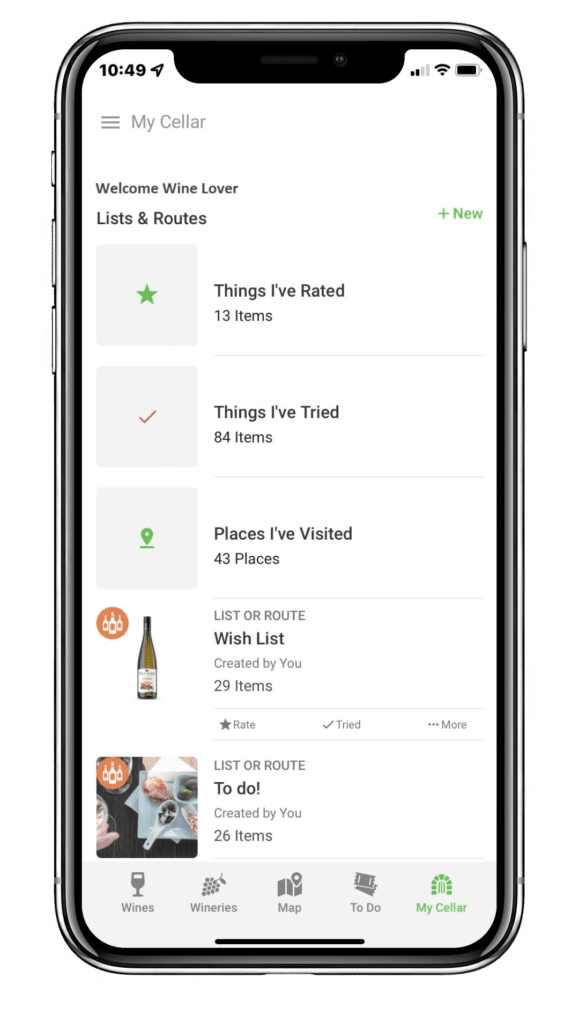The image is a photograph of a smartphone displaying a wine-related application interface, which could either be on an Android or an iPhone. The phone's screen reveals the power and volume buttons, the front-facing camera, and the microphones. In the top left corner, the time is shown as 10:49 with a small arrow icon indicating that location services are active. The top right corner displays the service, Wi-Fi, and battery icons, but the battery percentage is not visible.

Beneath this, the screen features gray text displaying "My Cellar." To the left of "My Cellar" is a menu icon represented by three horizontal lines. The app appears to be welcoming the user with "Welcome Wine Lover," suggesting that it is a wine enthusiast's application.

The interface includes sections labeled "Lists and Routes." The first list is marked with a star icon and titled "Things I've Rated," which contains 13 items. Following this, there's a checkmark indicator for a list named "Things I've Tried" with 84 items. Next is "Places I've Visited," listing 43 places. 

There's also a list titled "Wishlist created by you" with 29 items, indicated by a picture of a wine bottle with a small orange icon featuring three additional wine bottles. Another list titled "To Do created by you" shows 26 items and includes a top-down image of a plate of food.

At the bottom, a navigation banner presents options labeled "Wines," "Wineries," "Map," "To Do," and "My Cellar."